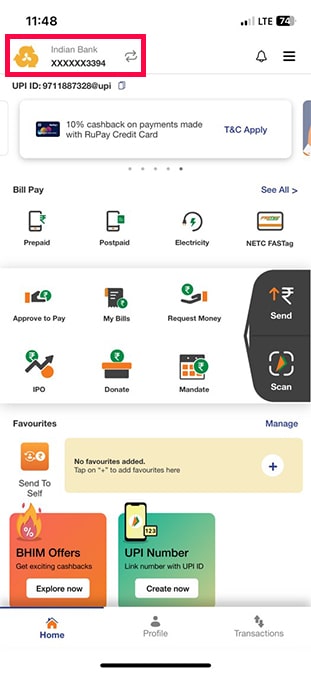A screenshot of a smartphone display captured and subsequently edited with a red box overlay is shown. The top right corner of the screen depicts a battery percentage icon at 74% and indicates an LTE connection with two bars of signal strength. The time in the top left corner shows 11:48. 

The red box, added post-screenshot via editing software such as Photoshop or Microsoft Paint, contains a three-arrow symbol followed by the text "Indian Bank XXXXXX3394" and a circular refresh/recycle icon. To the right of this, there is a bell notification icon and a three-bar menu icon.

Below this section, the text reads "UPID: 9711887328@UPI" accompanied by two paper icons. Further down, a white box highlights a credit card offer stating, "10% cashback on payments made with RuPay credit card. T&C apply."

The lower portion of the screen is populated with a variety of icons, each leading to different services. At the very bottom, three primary icons are visible: a home icon, a profile icon, and a transactions icon.